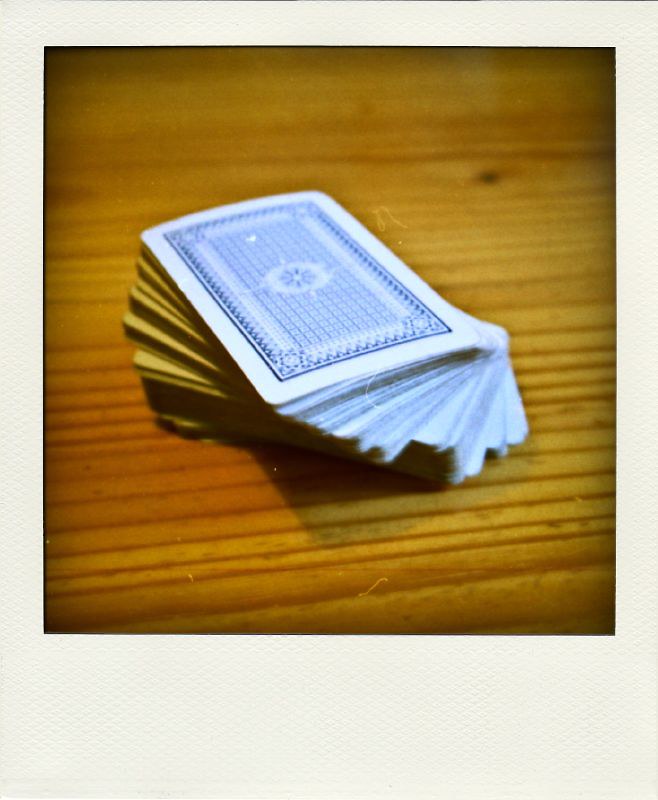This color photograph captures a neatly stacked deck of cards placed at the very center of a rustic, burnished wooden surface. The deck is slightly fanned out to the right, suggesting that someone has gently twisted it to achieve a decorative effect. The visible cards feature a striking blue and white intricate pattern reminiscent of designs found in Persian rugs, bordered by a series of ornate frames. Each card showcases a central flowery motif. The entire image is surrounded by a classic white Polaroid frame, adding a nostalgic touch with its thick, matte cardstock material.